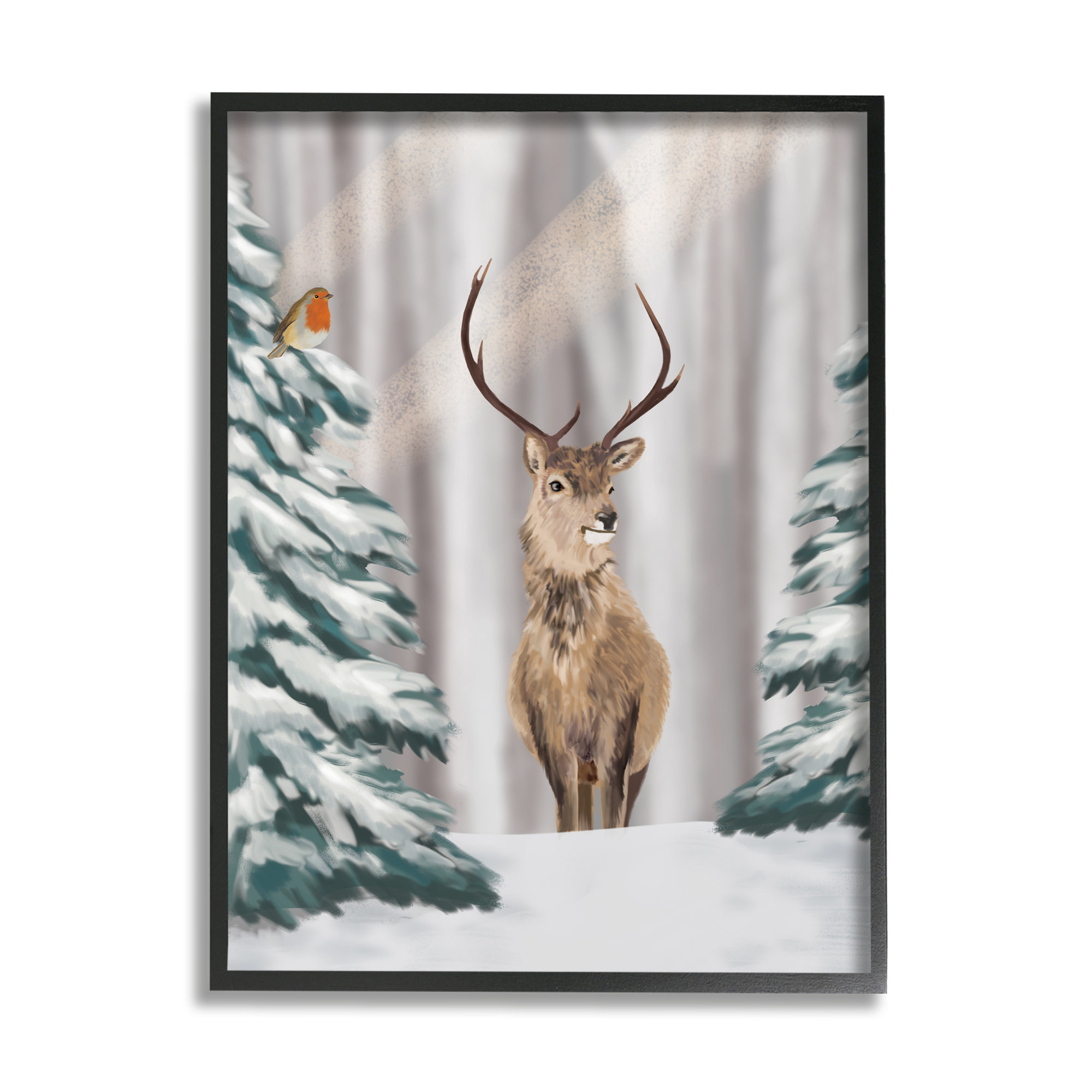In the image, framed with a black border, a serene winter landscape is depicted in the form of a detailed painting. The scene features a central deer, likely a buck, standing between two partially visible evergreen trees that resemble Christmas trees, their branches laden with freshly fallen snow. The deer, with a beautiful light brown coat and variations of darker brown on its legs and under its chin, has striking features including a white area around its mouth, a black nose, and black eyes that convey a subtle, almost content expression. Its impressive antlers majestically crown its head as it gazes to the left.

Perched atop the tree on the left is a small bird, possibly a robin, characterized by its orange belly and face, with a white section further beneath. The bird’s wings and beak are brown, and it too seems to have a gentle, cheerful demeanor. The background of the image is somewhat abstract, with blurred elements and stray rays of light enhancing the ethereal atmosphere. The overall artwork is rendered with fine brushstrokes reminiscent of an oil painting, capturing the tranquil beauty of this wintry woodland scene.